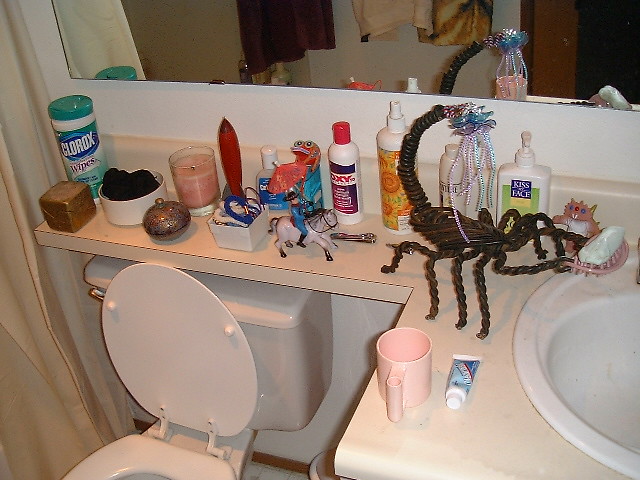In this rectangular photograph with a horizontal orientation, the primary focus is a bathroom countertop. The countertop, in a whitish-cream color, hosts an array of various items and takes up much of the frame. On the bottom right, a white sink is partially visible, while on the bottom left, there is a cream-colored toilet with its lid open but the seat down. The background features a white wall extending behind both the countertop and toilet. A large mirror is positioned above the countertop, though it is cut off at the top of the frame, making the mirror only partially visible. 

To the far left of the image, a golden curtain hangs down. The countertop itself is cluttered with numerous items: a bottle of Clorox wipes on the far left, a golden box, a white bowl, a decorative ornate oval box that might be intended for jewelry, and a pink candle. There is also an object resembling a small rocket standing up, a product labeled "oxy," a figurine of a man riding a horse, a bar of soap, and a pink cup. Additionally, a tube of an unidentified product is lying facing the camera, alongside a large, scorpion-like stand that seems designed for hanging necklaces or other accessories. Metal toenail clippers are also seen amidst the clutter.

The myriad objects offer a glimpse into the utilitarian and personal nature of the space, highlighting both cleanliness products and personal adornments side by side.